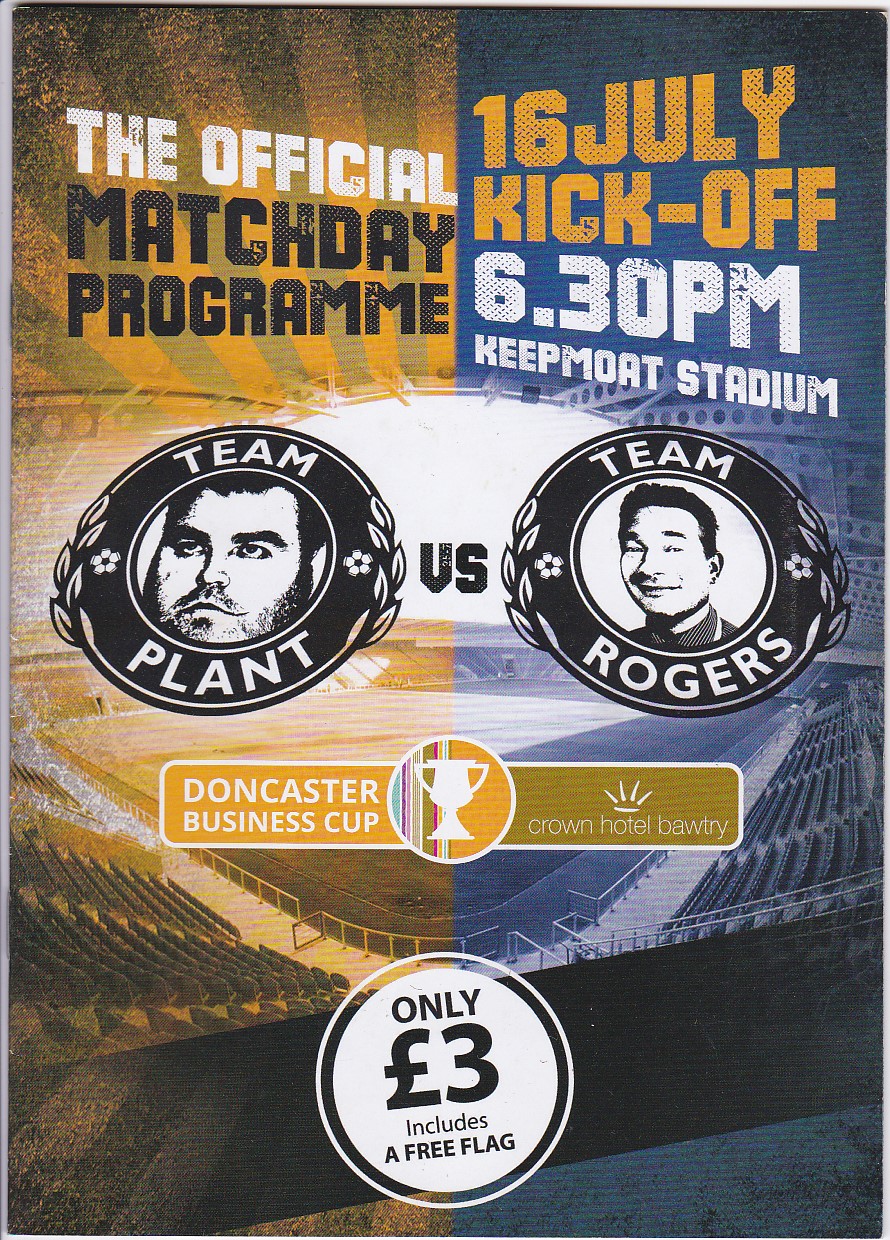This image is a detailed poster for a sporting event, visually divided into two halves with distinct color schemes–an orange background on the left and a blue background on the right. The background features a photo of a nearly empty sports stadium, tinted differently on each side.

On the left half, in white text, it reads "The Official" and below that in black, "Match Day Program." There is a prominent black circle with white text around its edge that reads "Team Plant." Inside this circle is a close-up black-and-white image of a man's face. Below this, "Don Caster" is written in white on a yellow background.

The right half of the poster highlights event details in vibrant colors: "16 July" in orange, and "Kickoff, 6:30 p.m." in white underneath. This information is followed by "Keep Moat Stadium." Below, another circular image features "Team Rogers" in white lettering on a black circle with a black-and-white portrait of a man's face in its center. Beneath this, against a beige background, is the text "Crown Hotel Ballery" in white. Centrally positioned at the bottom of the poster is a white circle containing black text that reads, "Only Three Pounds — Includes a Free Flag."

Floral and leafy decorations adorn the circular team images, adding aesthetic detail. In addition, in the middle, there is a silhouette of a trophy, emphasizing the competitive nature of the event.

This poster effectively combines vivid colors, essential information, and engaging graphics to promote an exciting upcoming matchday.